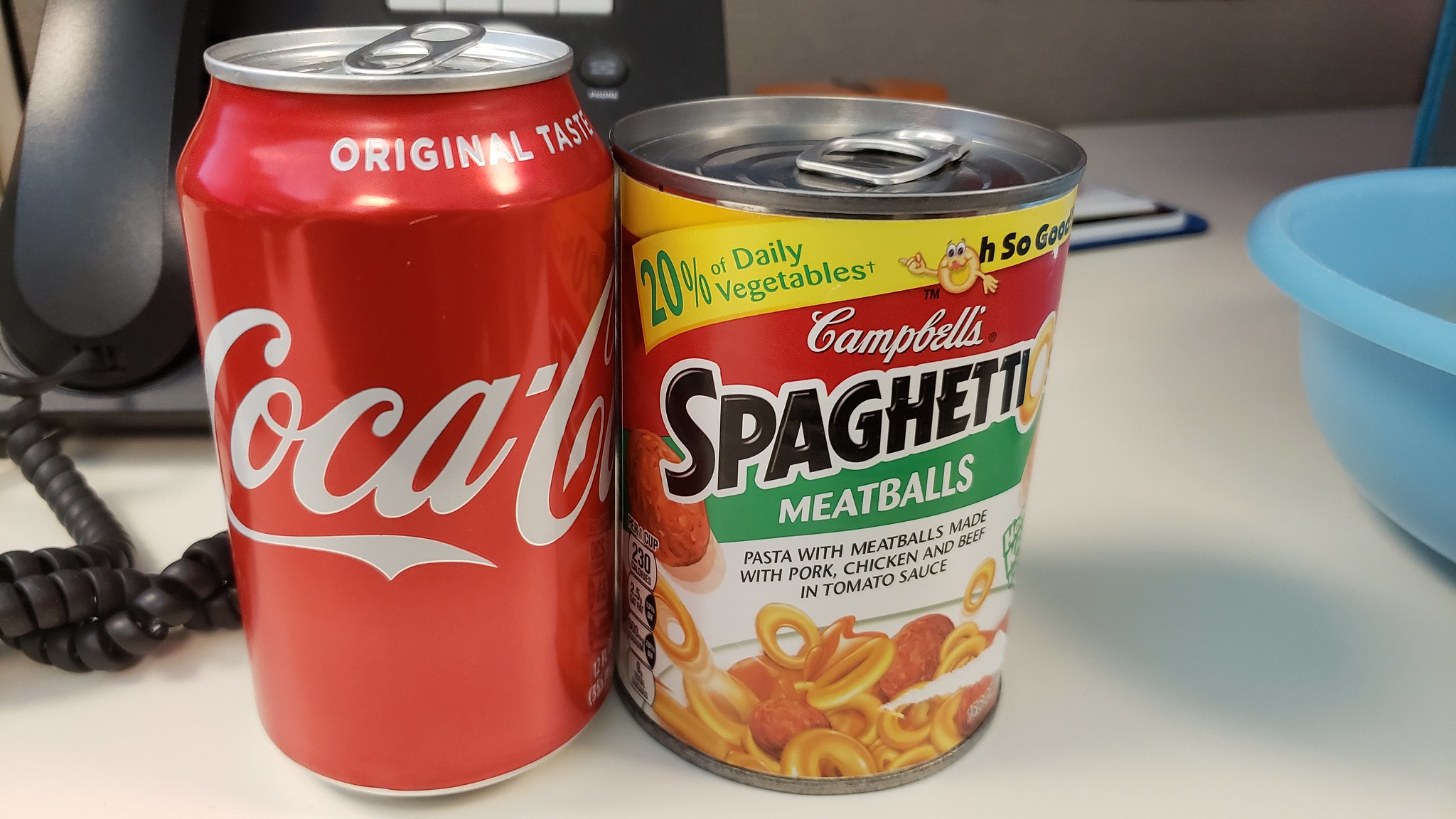A detailed image showcases an arrangement on what appears to be a desk, indicated by a traditional corded telephone in the background. Prominently featured in the foreground is a red can of Coca-Cola, adorned with the iconic white cursive logo, which appears to have been opened. Sitting directly next to it is an unopened can of Campbell's SpaghettiOs with Meatballs. The SpaghettiOs can boasts vibrant illustrations, including a depiction of pasta with meatballs in tomato sauce at the bottom, and informative highlights such as "20% of daily vegetables" on a small banner at the top. Adding to the scene, a blue bowl is visible near the cans, suggesting it may serve as the dish for the SpaghettiOs. The setting exudes a casual, everyday ambiance, with attention to both the familiar branding and the practical use of the items.